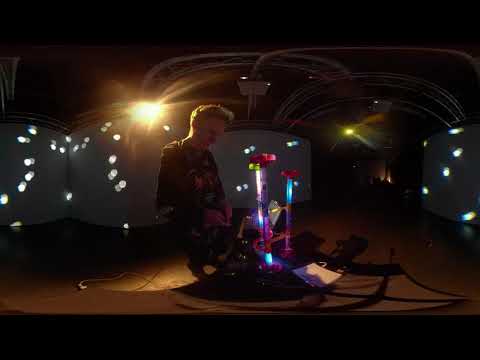In a dimly lit room with stark contrasts of light and shadow, a man, possibly Caucasian with short light hair, stands on a dark brown floor. He dons a black jacket, a black shirt adorned with planets, black pants, and black shoes. His gaze is directed downward towards an intricate contraption situated to his left. This device features two interlinked towers, both capped with red tops, and connected by a series of vibrant purple and orange tubes. The left tower showcases a gradient from purple to red, while the right transitions from blue to purple to red. The man's light-colored hands suggest he may be wearing a headset, adding to the scene's high-tech ambiance.

The backdrop is a white wall illuminated by an array of white lights projected from the ceiling. The ceiling itself is shrouded in darkness, save for several white tubes and a central white square projector. The right part of the scene reveals an open hallway and additional walls, both accented by more yellow and orange lighting. The overall effect is a blend of high-tech elements and striking visual distortions, with the proportions of the man and the device appearing elongated and bent. This captivating environment suggests an auditorium stage, enhanced by reflective screens both in front of and behind the man, creating a space filled with dynamic and colorful light interactions.